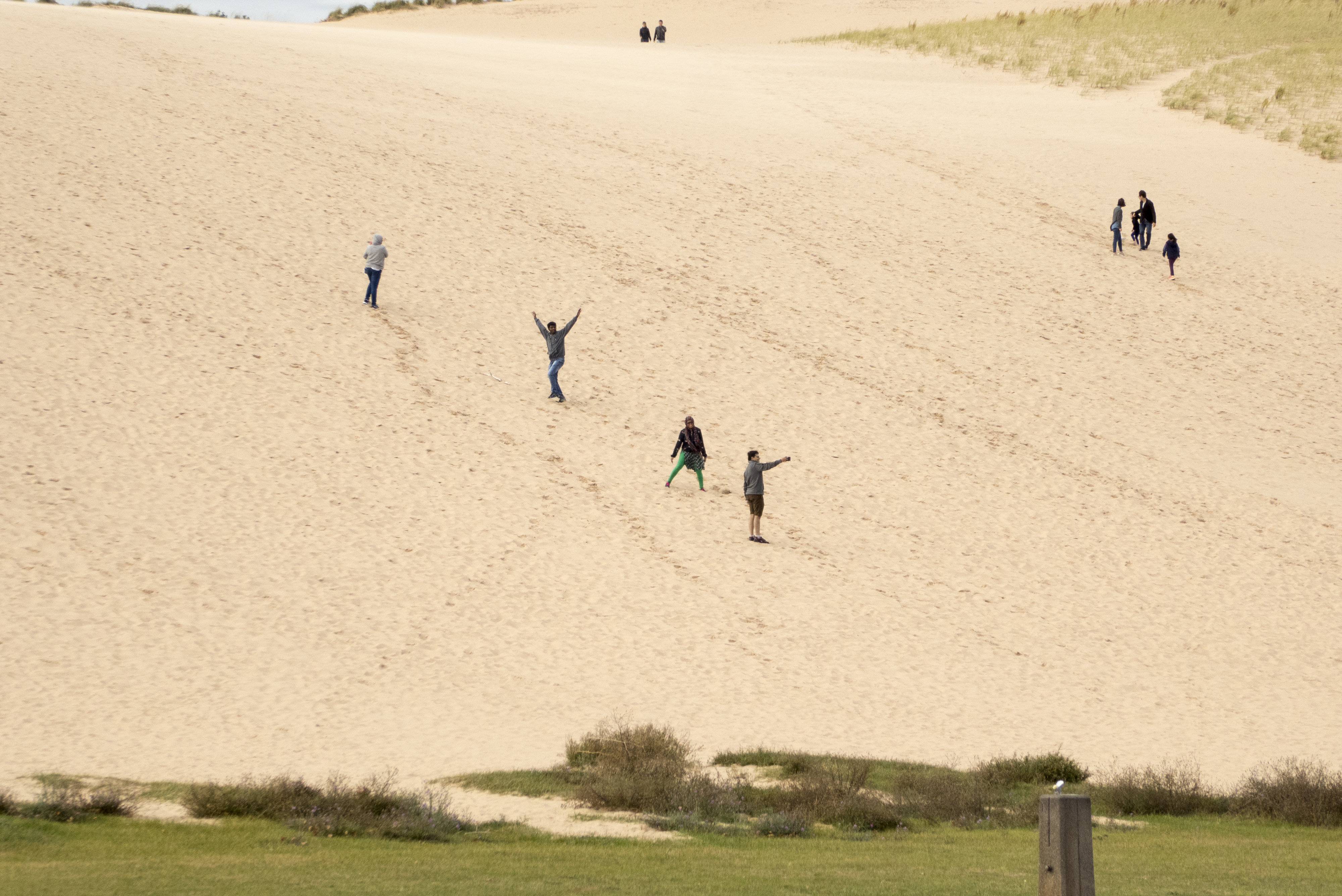The image is a color photograph captured from the base of a large sand dune, which stretches diagonally from the left to the right. The foreground showcases a patch of green grass interspersed with small bushes and a wooden pole. Up the sandy hillside, a group of nine people is scattered. At the base, a cluster of four individuals appears jubilant, turning back with hands raised, possibly celebrating. To their right, three more people are ascending the dune, seemingly headed toward a small sliver of water visible in the top left corner. At the very top of the dune, two figures stand, perhaps taking in the view, with patches of grass surrounding them. The overall scene captures the playful and dynamic ascent of the group against the expansive, sandy backdrop.